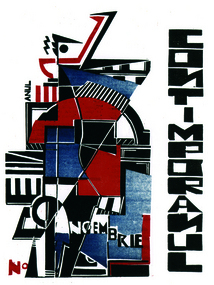The image depicts a bold and modern piece of abstract art characterized by a complex mosaic of various shapes and colors. Dominated by a palette of reds, blues, blacks, and whites, the artwork features an array of geometric figures, including stripes, rectangles, triangles, and half-circles, layered intricately upon each other. Prominently, vertical black and white letters cascade down the right side of the piece, spelling out "C-O-N-T-I-M-P-O-R-A-N-U-L" in chunky, boxy font, with each letter stacked below the previous one. Within the composition, more letters are visible; across the bottom, the sequence "N-O-E-M-B-R-I-E" is integrated into the design, not superimposed but seamlessly part of the image itself. Additional text appears in the left corner with an "N" followed by a small "O." The top section of the artwork seems to include an eye and a beak-like form, further enhancing its modernistic and avant-garde appeal. The artwork is layered and forward-facing, intended to evoke a sense of confusion and complexity in the viewer, highlighting its daring and abstract nature.